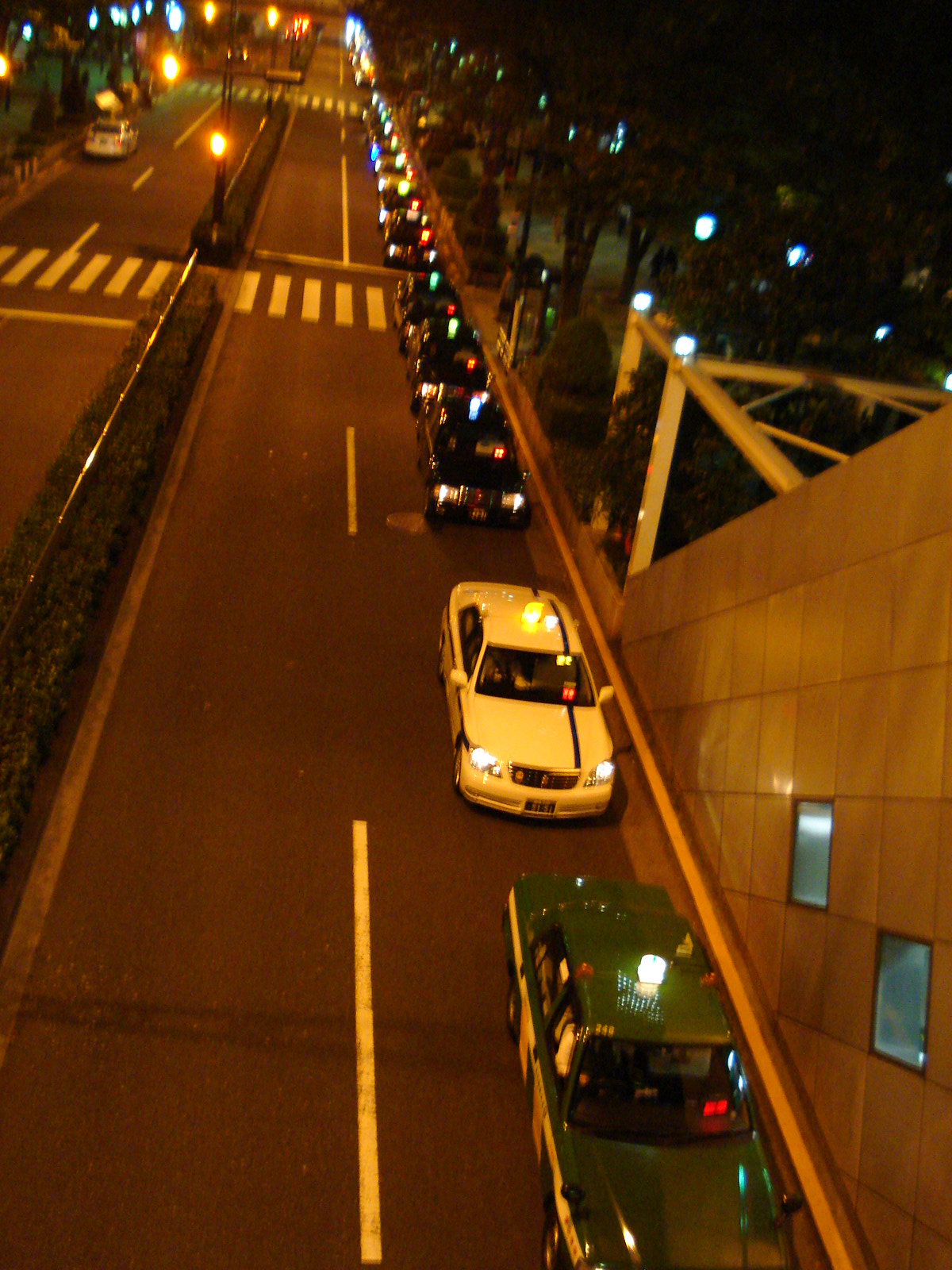A nighttime street scene features a two-lane road divided by a green hedged median with a shiny metal divider. The road has white rectangular lines marking the middle, and two crosswalks similar to those on the Beatles' Abbey Road album. On the right side of the street, a long line of cars, possibly taxis, with their bright white headlights on, appear to be in a traffic jam. These cars are of different luxurious colors, including green, black, and white, and are angled towards the perspective of the photographer, implying the photo might be taken from above. The left lane, heading in the opposite direction, is mostly empty except for a single white car. In the background, there is a steep hill and a silver, diagonally positioned modern building with two windows, adding to the scene's depth. Green trees and bushes are visible in the top right, blending with the urban environment. The photo, bathed in low light, creates a slightly glary and blurry effect, enhancing the nighttime atmosphere.